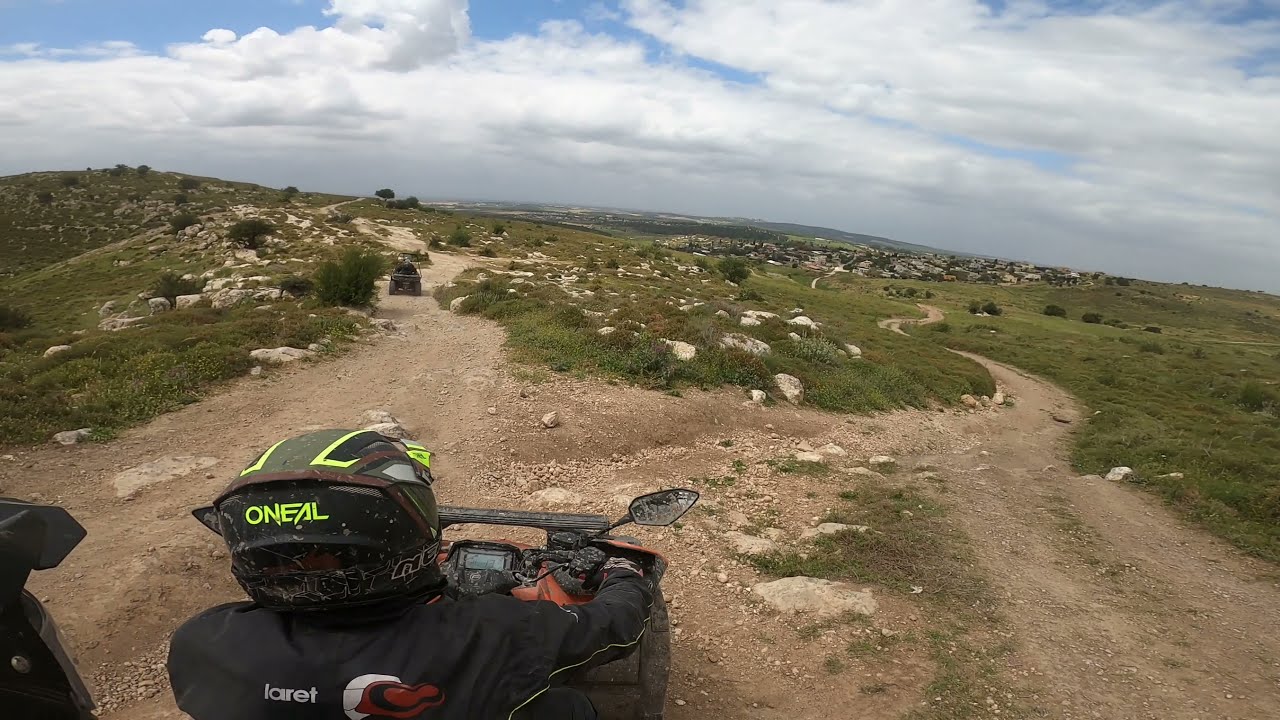In the foreground of a vast, outdoor landscape, a person rides an orange ATV with black wheels. The rider wears a black long sleeve shirt, black and white gloves gripping the handlebars, and a black helmet adorned with yellow stripes and font. The sky above is light blue with thick white clouds, while the terrain below features hilly, green landscapes interspersed with various rocks. The ground immediately beneath the ATV is a patchwork of brown dirt paths and rocky patches, which weave through the hills into the distance, surrounded by more greenery and a mix of white and gray rocks. A small mirror is visible on the vehicle, suggesting a rugged journey ahead through this expansive natural setting. The overall scene combines the vibrancy of the rider and their vehicle with the tranquil, contrasting elements of the landscape.